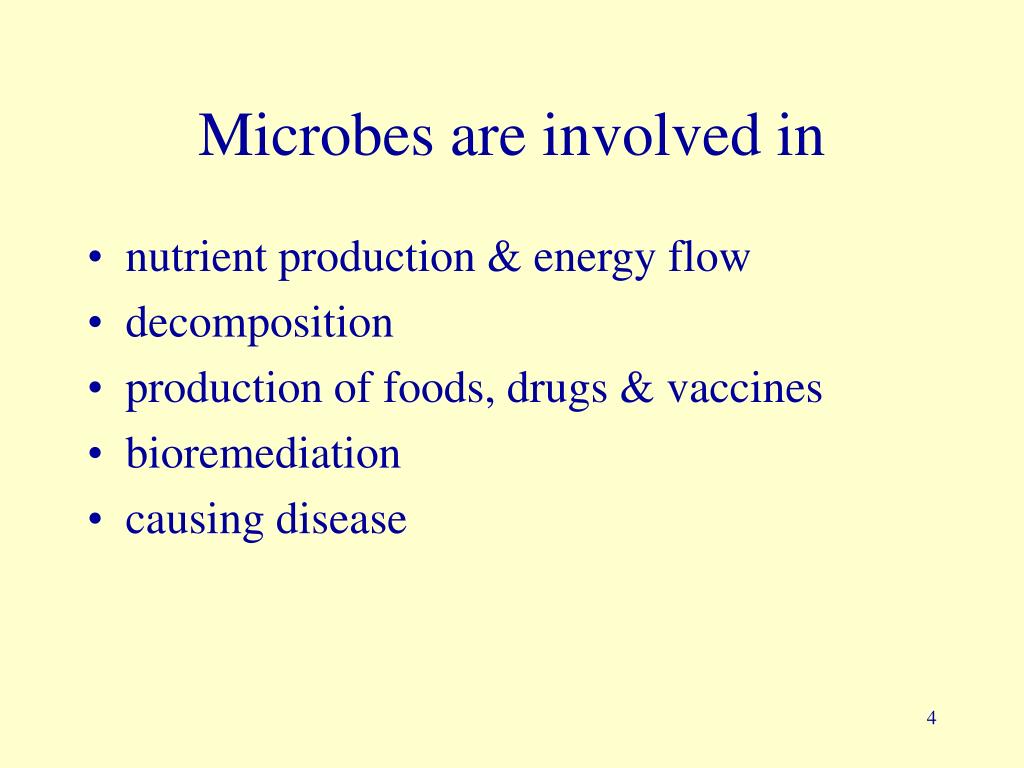This image appears to be the fourth slide in an educational PowerPoint presentation, featuring entirely text on a yellow background. Centered at the top in blue font is the title "Microbes are involved in." Below the title, aligned to the left, are five bullet points also in blue text: "Nutrient production and energy flow," "Decomposition," "Production of foods, drugs, and vaccines," "Bioremediation," and "Causing disease." The bottom right-hand corner displays a blue numeral "4," indicating this is likely the fourth slide in the series. The overall layout suggests the slide is designed to provide an overview of the various roles that microbes play.